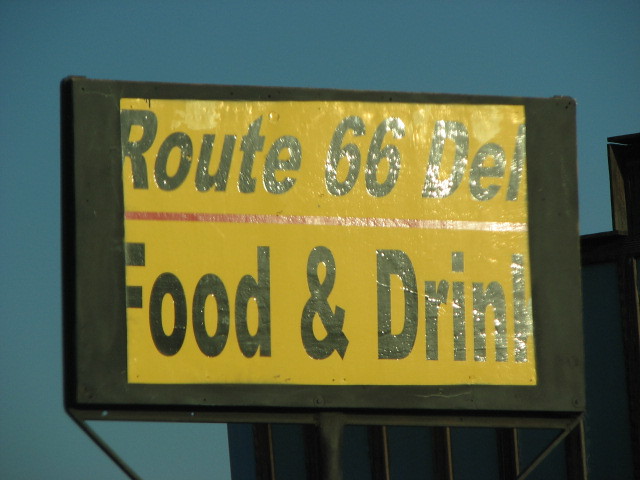The image captures a billboard-style sign prominently featuring a yellow rectangle with bold black italicized text that says "Route 66 DEL." The sign is bisected by a horizontal red line, beneath which the words "Food and Drink" are displayed in regular bold black letters. The sign has a black border and is mounted on a black rod that extends downward, out of the frame. The right edge of the sign seems slightly truncated, possibly cutting off some text. The photo appears to have been taken at an angle and includes reflections on the sign's surface, indicating bright sunlight. In the background, there's a clear, slightly dark blue sky without clouds, and the black reverse side of another sign is visible at the bottom right corner of the image.